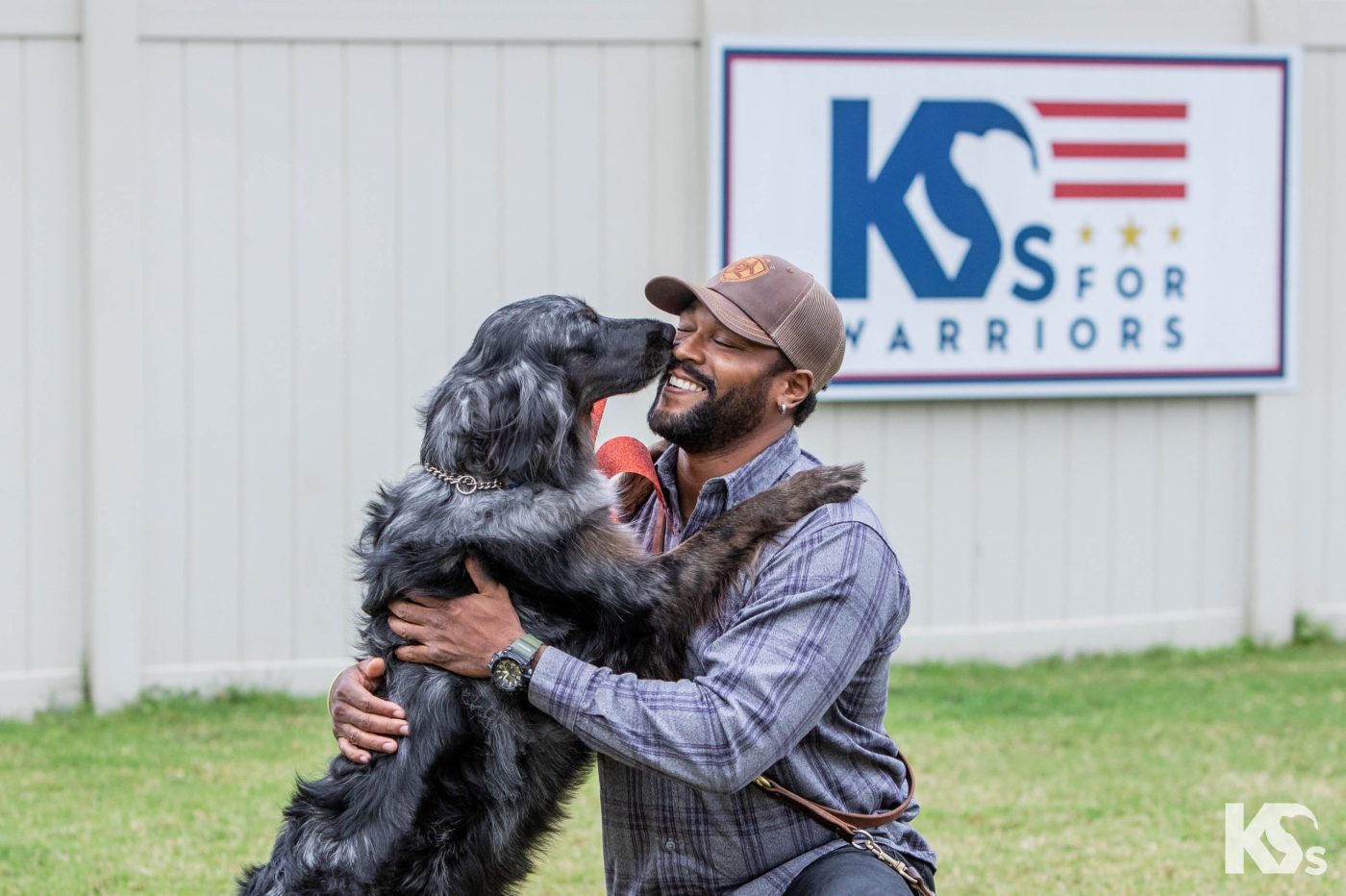In this vibrant, colored outdoor photograph taken during the day, an African-American man is showcased in a three-quarter view, kneeling down and warmly embracing a large black Labrador, which has white and gray streaks in its long, slightly shaggy fur. The dog, wearing a chain collar and leash, stands on its hind legs with its two front legs resting on the man's shoulders, affectionately licking his nose and making direct eye contact with him. The man, who sports a closely shaven beard and mustache, smiles with his eyes closed. He is dressed in a blue checkered shirt, blue jeans, a brown trucker's baseball cap with an orange patch, and a black watch with a green band on his left wrist. Behind them is a white picket fence adorned with a prominent sign reading "K9s for Warriors," which is bordered by a blue outline and embellished with three red stripes and three gold stars. A logo in the bottom right corner of the image mirrors the "K9s" text along with a dog silhouette. The scene exudes a sense of companionship and joy, set against a backdrop of green grass and a supportive message for a service dog organization.